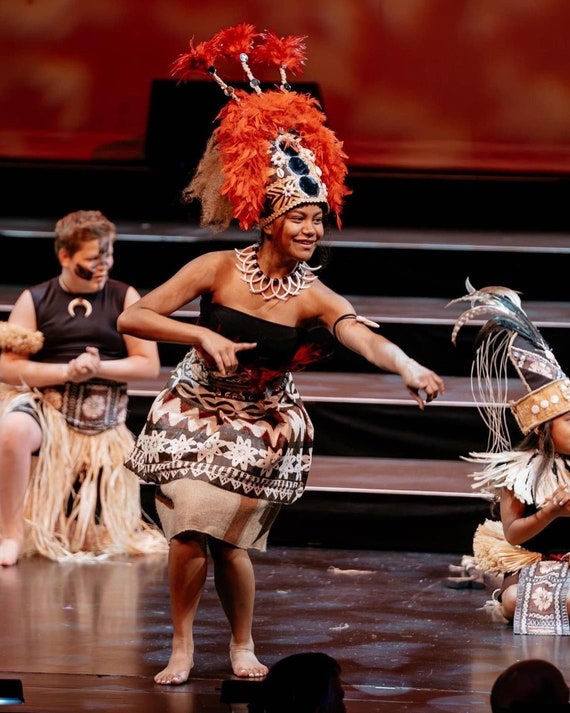The image features three individuals on a stage, partaking in what appears to be a cultural dance or celebration. The focal point is a preteen or teenage girl with darker skin, dressed in an elaborate outfit: she wears a large, intricate headdress adorned with jewels and red-orange feathers, a sleeveless dress covered in various designs, a patterned skirt, and a striking necklace made of long, white teeth or bones. She is barefoot and has white powder make-up on her feet and arms, accompanied by a bracelet on her upper arm.

Behind her, a seated younger individual, also dark-skinned, sports a similar tall feathered headdress and a feathered collar. To the left, a teen boy with face paint and a black sleeved shirt complements his look with a grass skirt over his pants. All three are dressed in outfits suggesting an indigenous or Polynesian cultural celebration, possibly with influences resembling Maori or Hawaiian traditions. The stage, with visible steps in the background and the heads of audience members seen from behind, sets the scene for this vibrant performance.